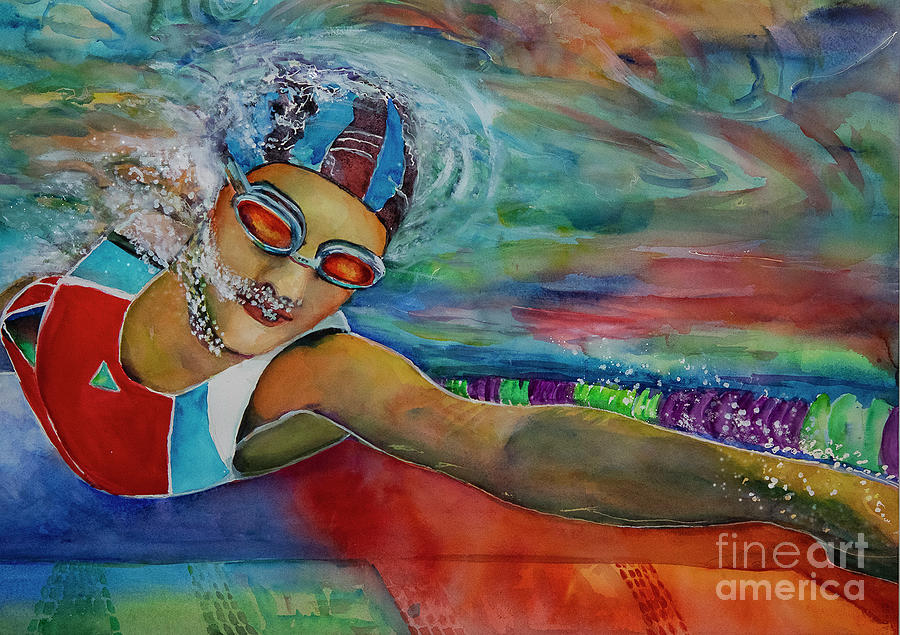This is a detailed underwater painting of a woman swimming competitively. She is depicted with a dark complexion and a focused expression, indicating her competitive nature. She wears a blue and black striped swim cap and amber-colored swim goggles with orange lenses. Her one-piece bathing suit is primarily white, blue, and red, with some green accents. The suit's blue and red colors are most prominent on the front of her chest, with white on her shoulders. Her left arm is outstretched, extending out of the frame at the bottom right corner, and she is swimming towards the artist's point of view.

Bubbles are visible, streaming from her mouth and nostrils, and creating a dynamic sense of movement as they float towards the surface of the water, which is visible above her. Additionally, there are droplets of water coming off her chin, enhancing the realism of the scene. The painting's background features multicolored, swirling patterns reminiscent of a watercolor style due to the bleeding of colors into one another. In the bottom right corner, there is a faint watermark that reads, "Fine Art America."